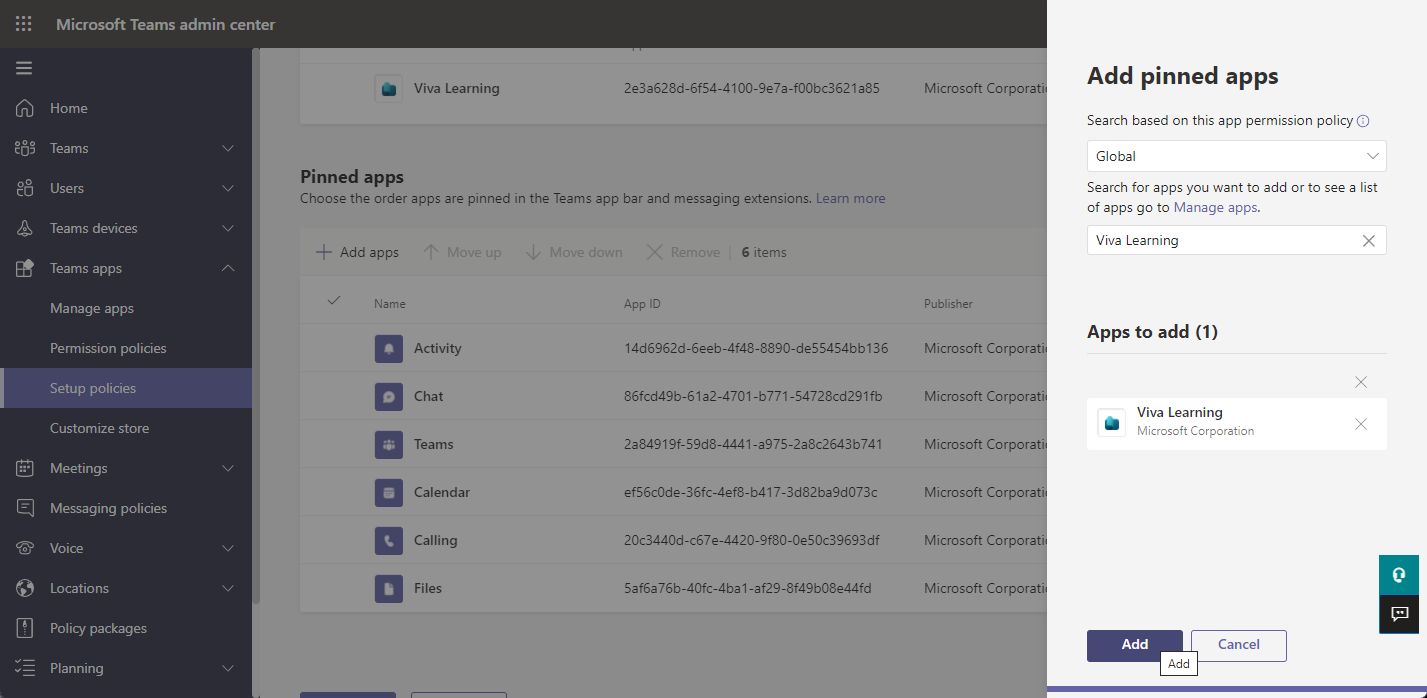Detailed Caption: 

The image depicts a screenshot of the Microsoft Teams Admin Center interface, with dimensions roughly 50% wider than it is tall. The layout is predominantly grayed out, creating a haze that visually separates the primary window on the right from the rest. 

In the upper left corner, there's a grid of white dots set against a black background bar, adjacent to which the text "Microsoft Teams Admin Center" is displayed, extending over 75% of the image's width.

On the left side of the interface is a vertical navigation menu, featuring icons and text labels in white over a black background. This black background ends approximately 20% into the image. The menu includes the following options from top to bottom:
1. Home
2. Teams
3. Users
4. Teams devices
5. Teams apps
6. Manage apps
7. Permission policies
8. Setup policies
9. Customize store
10. Meetings
11. Messaging policies
12. Voice
13. Locations
14. Policy packages
15. Planning

To the immediate right of the navigation menu lies the "Pinned apps" section, which continues into the main window occupying the right quarter of the image. This section lists various apps, represented with purple icons. 

In the main window on the right, the heading "Pinned apps" is prominently displayed. Below this, a search field is available, captioned with "Search based on the app permission policy." A drop-down box has been selected to show the global setting.

Overall, the image captures the streamlined interface of the Microsoft Teams Admin Center, highlighting its navigation options and pinned apps management area.